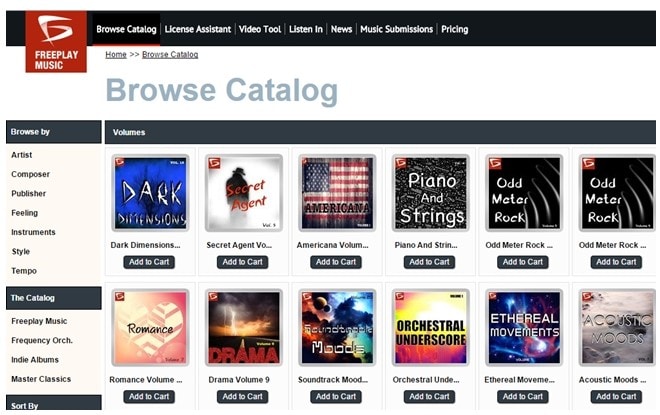Screenshot of the Freeplay Music Website:
 
The image is a horizontal screenshot of the Freeplay Music website, captured from a computer. The absence of a taskbar or search bar suggests it focuses solely on the website content. 

At the top left corner, the distinctive Freeplay Music logo is prominently displayed. The logo features white lettering and an emblem that artistically blends the letters "F" and "P" on a red square background.

Running horizontally across the top of the webpage, there is a black navigation bar with white text, offering various options. The available options include 'Browse Catalog,' 'License the Assistant,' 'Video Tool,' 'Listen In,' 'Music Submissions,' and 'Pricing'. The 'Browse Catalog' option is currently selected, as denoted by the breadcrumb-like trail below it: "Home > Browse Catalog > Browse Catalog" in large letters.

Situated on the mid to bottom left of the screenshot is an extensive menu to refine the browsing experience. Users can navigate by 'Artist,' 'Composer,' 'Publisher,' 'Feeling,' 'Instrument,' 'Style,' or 'Tempo'. Additionally, users can choose from different catalogs such as 'Freeplay Music,' 'Frequency,' 'Orchestra,' 'Indie Albums,' and 'Master Classics'. A 'Sort by' option exists but is cut off from the screenshot.

The main body of the screenshot showcases the search results under 'Browse Catalog,' revealing a variety of music volumes. Titles visible include 'Dark Dimensions,' 'Piano & Strings,' 'Ethereal,' 'Acoustic,' 'Orchestral,' 'Soundtrack,' and 'Drama.'